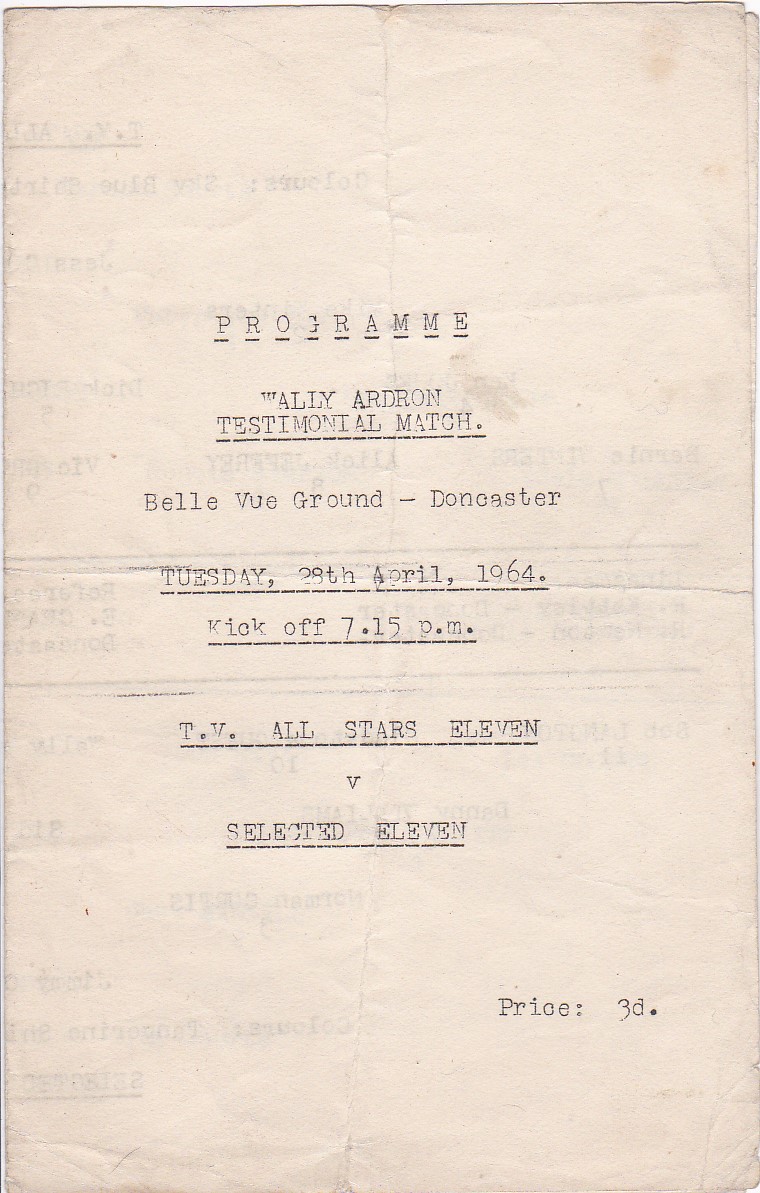The image depicts an aged and well-used black-and-white program cover for a testimonial match. The paper, now yellowed and stained with time, seems to have been folded multiple times, and the ink appears slightly runny and faded. At the top, the word "PROGRAMME" is prominently underlined. Below, it reads "Wally Ardron Testimonial Match" at the Bellevue Ground in Lancaster, scheduled for Tuesday, 28th April 1964, with a kickoff time of 7.15 p.m. The match is between "TV All Stars XI" and "Selected XI," with the program priced at 3d. There are no illustrations or charts on the cover, only a simple, typewritten text that imbues the piece with a strong sense of nostalgia and history.